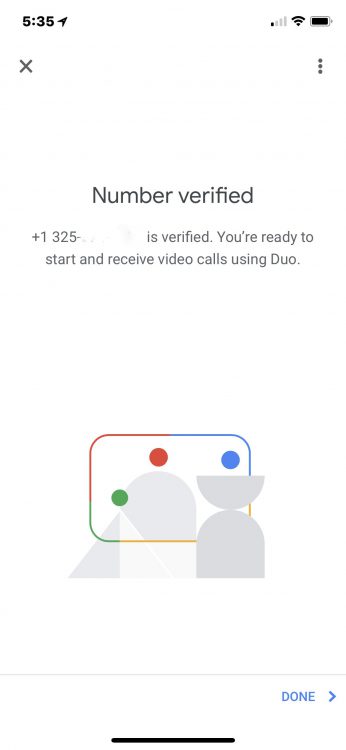This image is a screenshot from an Android phone displaying a confirmation message from Google Duo. At the top of the screen, the clock reads 5:35. The status bar shows various icons: a GPS navigation icon, a single bar of network signal strength out of four, enabled Wi-Fi connectivity, and a fully charged battery that is not currently charging. All icons and UI elements, including the clock, are rendered in flat black colors.

Below the status bar, there is an 'X' icon, likely used to exit the screen, and a three-dot menu underneath the battery icon for additional options. The primary message on the screen reads, "Number verified, +1 325 XXXX," with the rest of the phone number redacted. The message confirms that the user's number is verified and they are ready to start and receive video calls using Google Duo.

The image prominently features a Google Duo icon, characterized by Google's signature colors: green, red, blue, and yellow. The icon depicts a stylized figure with a rounded body and a semicircular head, staying true to Google's minimalist design ethos. At the bottom left corner of the screen, there is a button labeled "Done," likely to complete the setup process. This screen seems to confirm the successful verification of the phone number for using Google Duo's video calling services.